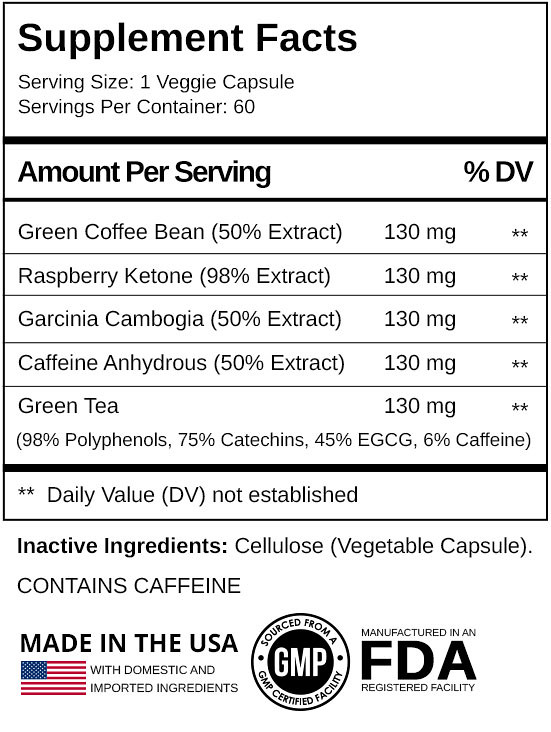This image displays the back label of a dietary supplement bottle. The label provides detailed information on the supplement facts, noting that each serving is one vegetable capsule, with 60 servings per container. The amount per serving includes:

- Green Coffee Bean Extract (50%): 130 mg
- Raspberry Ketone Extract (98%): 130 mg
- Garcinia Cambogia Extract (50%): 130 mg
- Caffeine Anhydrous (50% extract): 130 mg
- Green Tea: 130 mg

Directly below the supplement facts, the label lists the inactive ingredient as cellulose vegetable capsule. Additionally, in bold capital letters, the label emphasizes that the product "CONTAINS CAFFEINE."

At the bottom of the label, there are various certifications and origin statements. It proudly declares "Made in the USA" with an American flag illustration, noting the use of both domestic and imported ingredients. Adjacent to this, there is a symbol indicating the supplement is sourced from a GMP (Good Manufacturing Practice) certified facility, with "GMP" prominently displayed in the center of the emblem. Near this, it confirms that the product is manufactured in an FDA registered facility.